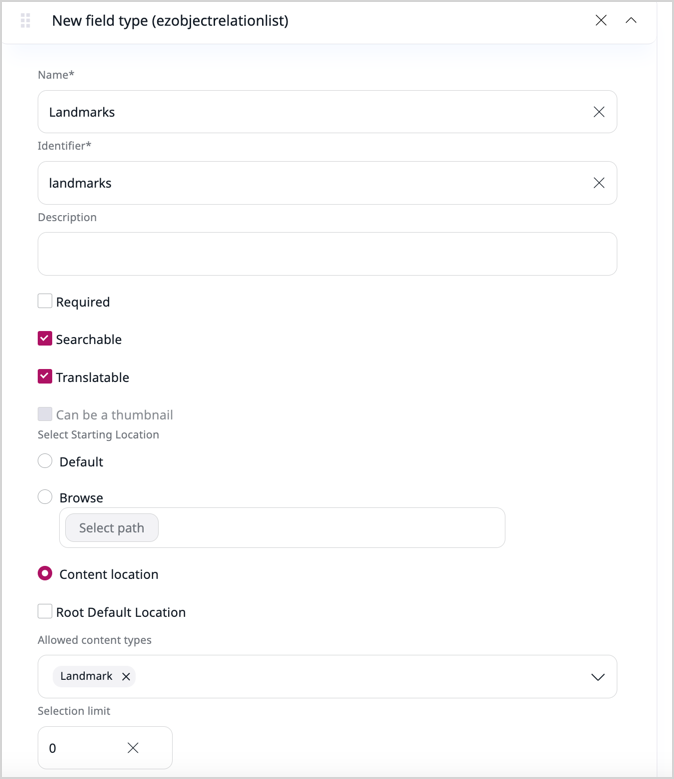The image depicts a user interface screen featuring various data input fields and options. At the top, there is a text identification label "ezobiectrrelationlist," though the correct spelling or meaning remains unclear. In the top right corner, there is an icon of a trash can symbol beside an arrow pointing downward.

Below this header, the screen contains several labeled sections:

1. **Name:** 
   - A blank field for entering the name of the item.

2. **Landmarks:**
   - **Identifier (Landmarks):** Another blank field for entering an identifier related to landmarks.
   
   - **Description:** A blank box provided for additional description.

   - **Options:**
     - **Required:** Accompanied by a checkbox, which is not checked.
     - **Searchable:** Accompanied by a checked checkbox.
     - **Translatable:** Accompanied by a checked checkbox.
     - **Can be a Thumbnail:** Accompanied by an unchecked checkbox.

3. **Category:**
   - A dropdown menu or selection box, which currently has "Content" selected.

4. **Location:**
   - **Select Location:** Next to this label is another blank box with a trash can icon beside it. 

5. **Allowed Content Types:**
   - In this section, "landmark" is listed. 

All text on the screen is predominantly in black, with some elements in gray, set against a white background.